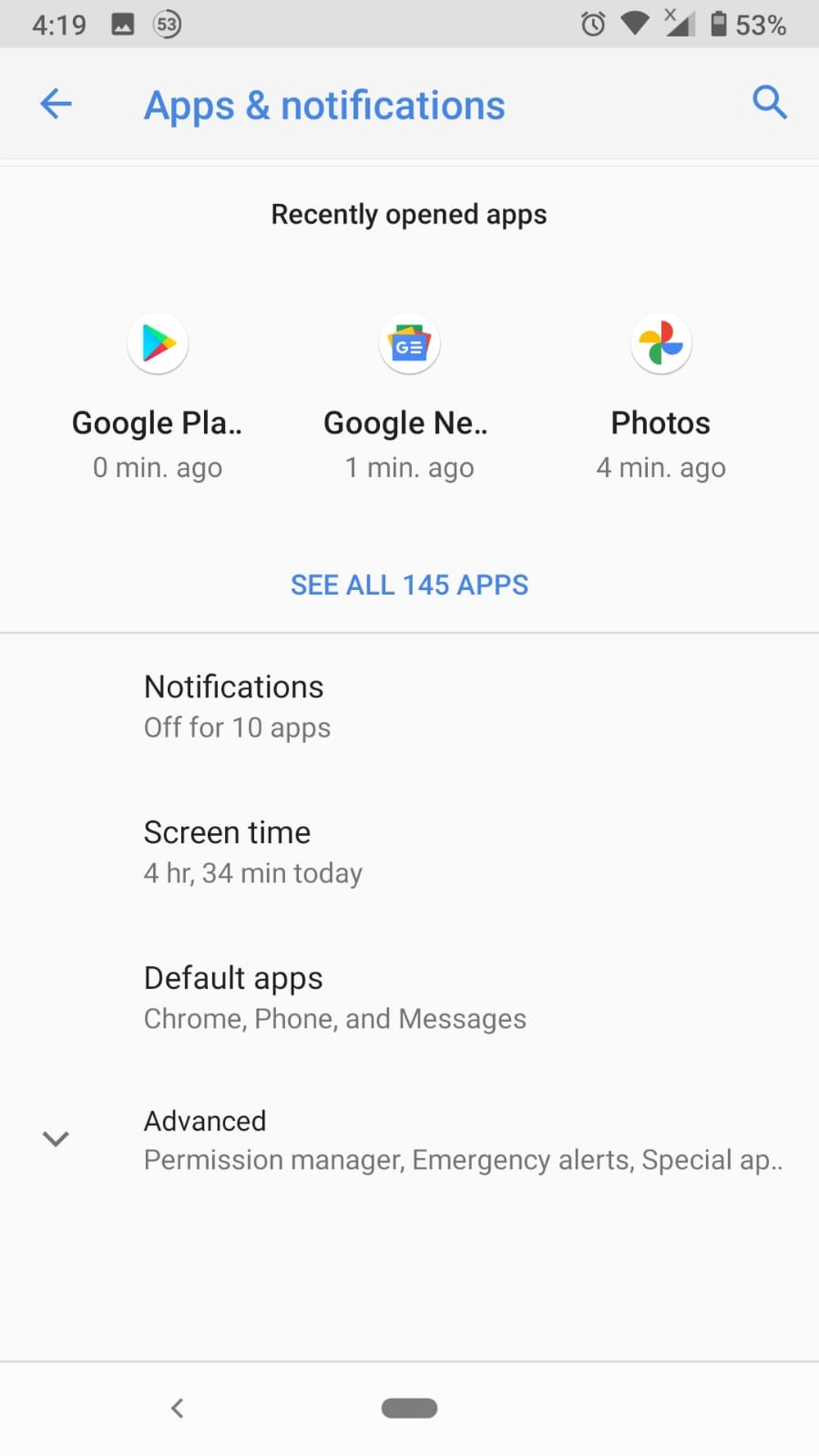**Detailed Caption:**

This image showcases a section of the settings interface on a mobile device, likely a smartphone or tablet. The layout is presented in a vertical format. 

At the top, there is a gray status bar indicating several icons and status notifications. On the upper-left corner, it displays the time "F419", accompanied by a photo icon and the number "53" encircled next to it. On the upper-right side, there are several icons: an alarm clock, a Wi-Fi signal indicator, a data icon marked with an "X" (indicating no data connection), and a battery status icon showing 53% battery life. 

Directly below this status bar, the background color transitions to a lighter gray. On this section, there is a blue left-facing arrow along with the text "Apps & notifications," accompanied by a blue magnifying glass icon. 

Below this header, in black font, is the section titled "Recently opened apps" with icons and names of recently accessed applications listed: Google Play, Google Any, and Photos. Just beneath this list, a blue clickable link reads "See all 145 apps."

Further down, additional settings are detailed in black text:
- "Notifications: Off for 10 apps."
- "Screen time: 4 hours 34 minutes today."
- "Default apps: Chrome, Phone, and Messages."
- "Advanced: Permission manager, Emergency alerts, and Special apps," which features a drop-down arrow suggesting more options can be expanded here.

At the very bottom of the screen, navigation options for the device are visible, including a button to return to the home screen and a back button.